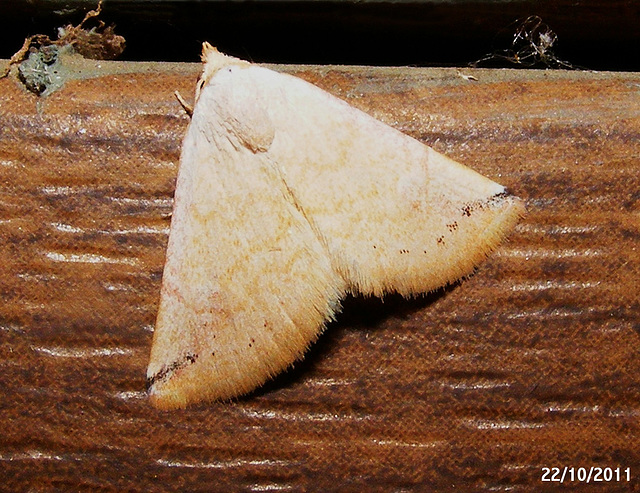This close-up photograph captures a small moth perched on what appears to be a piece of wood or an old book binding. The image is highly detailed, showing the moth's intricately patterned wings, which form a perfect triangular shape with a heart-like curve at the bottom. The wings display a gradient of colors, starting with a light, almost white tan near the head, and transitioning to darker tan and finally a dark brownish-orange at the tips. Dark brown or black specks can be seen towards the base of the wings. The surface on which the moth rests shows signs of age, with visible fibers, tattering, and what looks like water damage. The wood or binding appears dark brown and worn. In the bottom right corner of the photo, the date "22-10-2011" is clearly visible, adding a timestamp to this detailed and textured image.